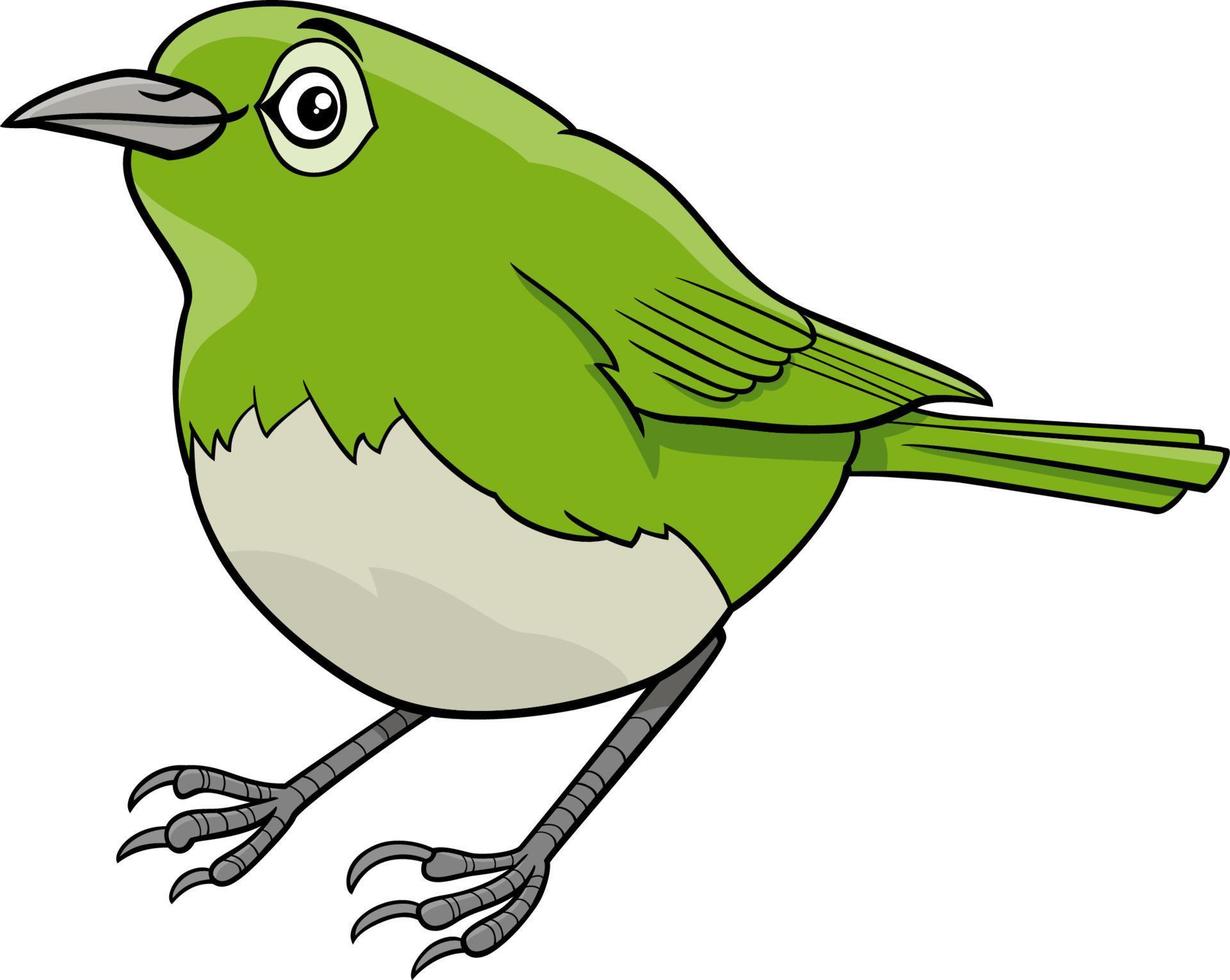A large cartoon drawing of a bird is presented in an outdoor setting, set against a solid white background with no border or text. The bird’s body is rather wide, with the upper half—including the wings, tail, and head—covered in medium green feathers, while the bottom half, comprising the belly and breast, is light gray. The bird has a long beak, also gray, that tapers to a point, and it faces left along with the bird's large eye, which features a black eyelid and pupil, a light green border, a detailed white interior with a smaller black circle, and a tiny white dot inside it, giving it a vivid, expressive look. The bird’s eye appears to be looking directly at the viewer and has a black eyebrow above it. The bird stands on two legs, each banded in darker gray and ending in three long claws. Its feet are positioned at an angle from right to left, not perfectly aligned with its body. Shadowing adds depth to the bird, particularly along the bottom of the belly, the tops of the legs, and the back of the tail. Only one wing is visible, tucked in and partially hidden. The tail is made up of three long feathers. Despite having no explicit smile, the bird’s overall demeanor seems friendly and inviting.